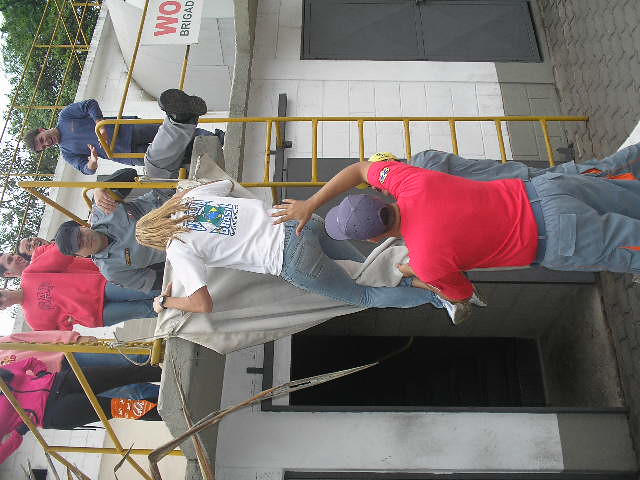The image, originally intended to be viewed in portrait orientation but shown horizontally, depicts a scene of multiple people engaged in what appears to be a construction or repair activity on a white concrete building with gray bottom and a yellow scaffold ladder. Central to the image is a woman with blonde hair, dressed in light blue jeans and a white t-shirt featuring some blue and green design on the back. She seems to be in the process of either climbing up or down from a platform, aided by a man in a red shirt, blue hat, and gray pants.

Above her sits a man in a gray uniform and blackish gray hat, with one black-shoed leg hanging off the platform. To his left, slightly behind, is another individual in a red sweatshirt and light blue jeans. Nearby stands a person in a pink jacket, black leggings, and an orange bandana tied around her right calf, her head out of frame. Further in the background, barely discernible, are two faces behind the person in the red sweatshirt.

Another man, dressed in a blue long sleeve shirt and black pants, stands on the far right side of the platform. Distinctly making the backdrop of this busy scene is a sign that reads "WO Brigade" affixed next to the yellow railing. Observations indicate that despite the presence of the yellow ladder, it is not being used by those climbing or aiding others on the structure. The collective atmosphere reflects a dynamic and cooperative effort, with numerous individuals, possibly workers, captured in various stages of action amidst a seemingly organized, group task.